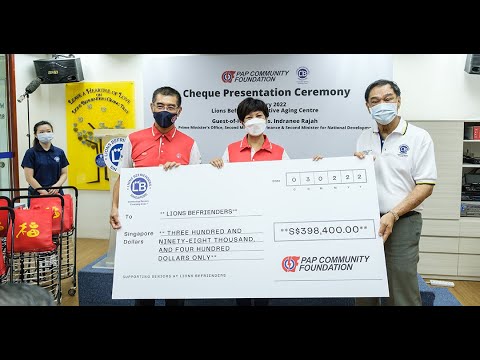The image depicts a detailed scene of a ceremonial check presentation indoors, with fluorescent lighting. Central to the photo, three Asian individuals in masks are prominently holding a large check. They are flanked by a fourth masked individual standing to the left. Behind them, a bold banner reads "Check Presentation Ceremony," alongside some illegible writing. The check, prominently displayed, is made out to "Lions Befrienders" for the sum of $398,400 and is issued by the PAP Community Foundation, a detail confirmed by visible logos on the check. The individuals holding the check include one man and one woman in red polos, and another man in a white polo. Nearby, a woman in a blue polo stands by shopping baskets adorned with red and gold tote bags featuring Chinese writing. On the top left of the image, a microphone and speaker attached to the wall indicate the formal nature of the event. The setting, marked by the British spelling "cheque," suggests it likely took place in a region where this variant is standard.